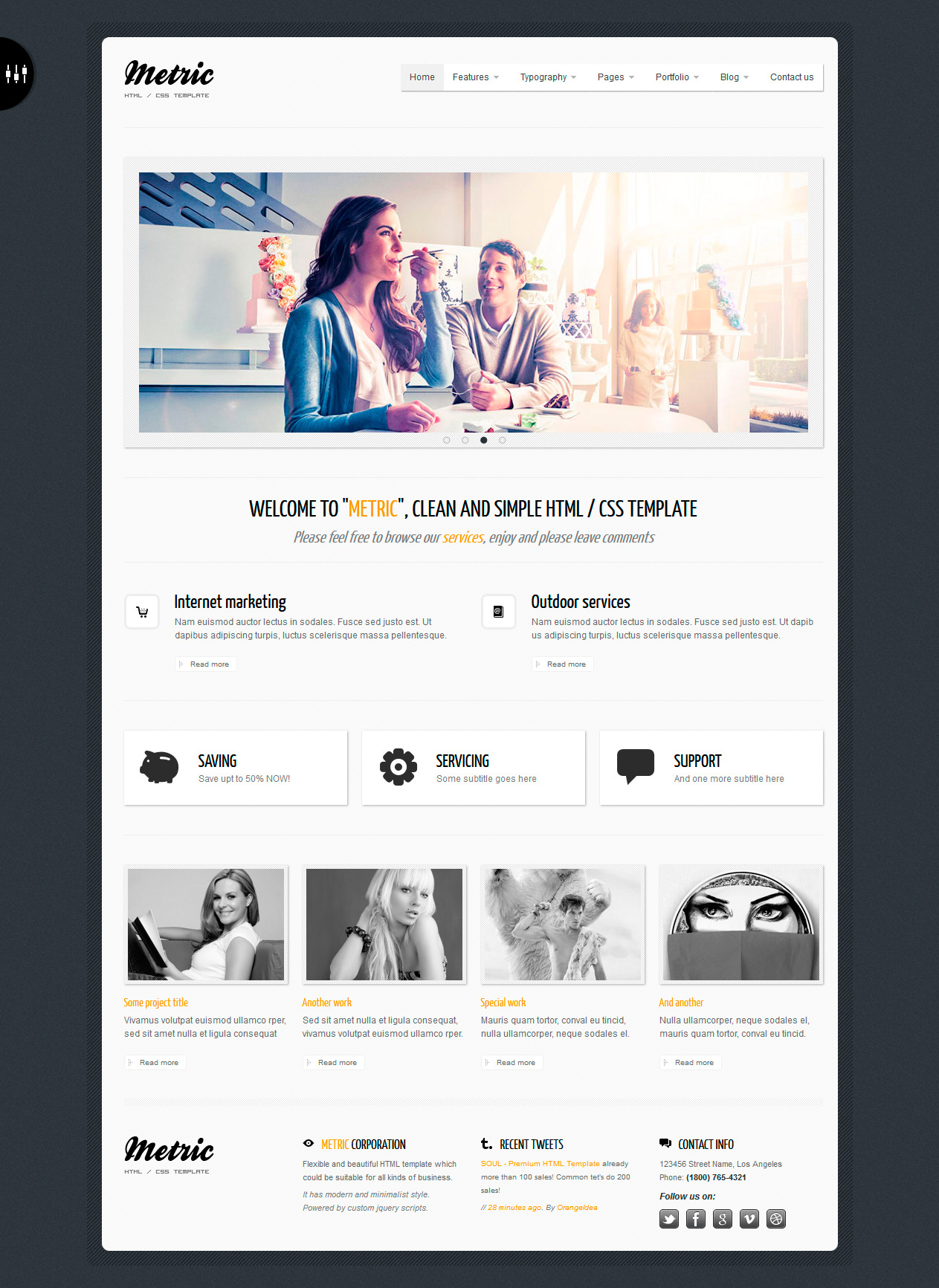A screenshot of a webpage titled "Metric HTML/CSS Template" features a well-organized layout with a navigation bar on the right, containing buttons for Home, Features, Typography, Pages, Portfolio, Blog, and Contact Us. Dominating the top section is a large image of a joyful woman in a blue shirt and white camisole, eating with a utensil in her mouth while smiling. A man beside her watches her with a smile, and a woman in the background, blending with the whitish-peach color scheme, gazes at them.

Beneath the main image, text welcomes visitors to "Metric Clean and Simple HTML CSS Template," inviting them to browse services, enjoy the content, and leave comments. The webpage offers an overview of various services, including Internet Marketing and Outdoor Services. Three distinct boxes highlight key offerings: Saving, Servicing, and Support.

Further down, the page showcases a series of four black-and-white thumbnail images, each labeled with project titles: "Some Project Title," "Another Work," "Special Work," and "And Another."